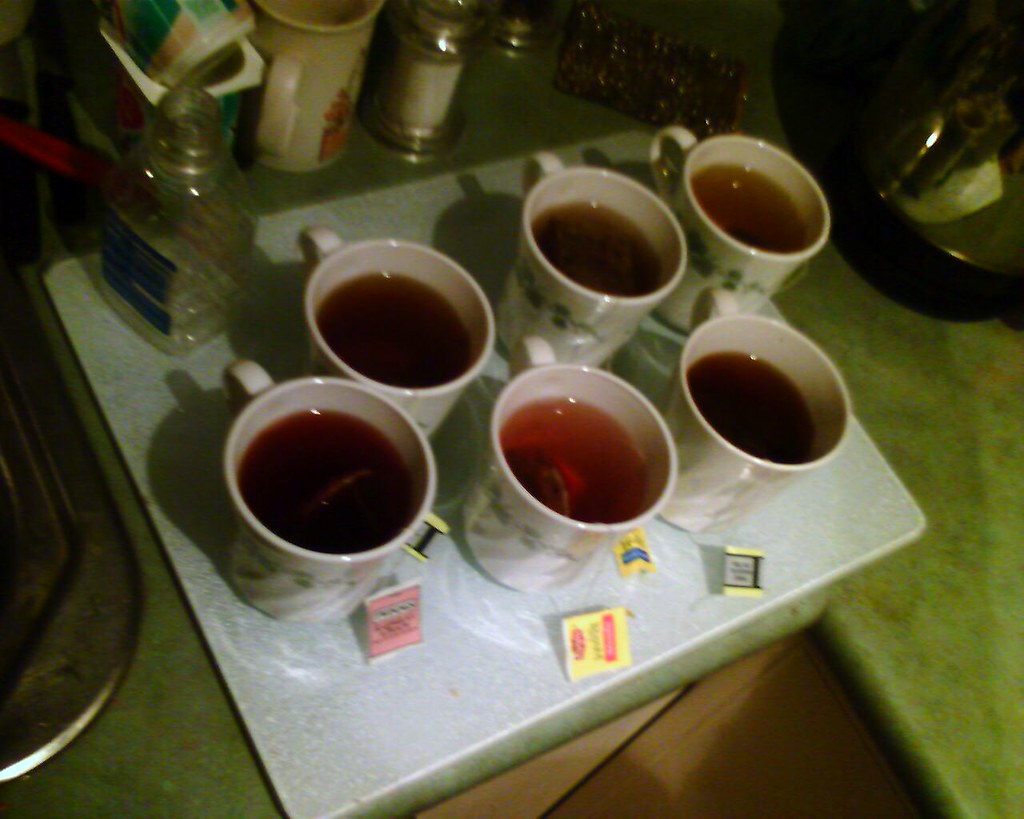This detailed digital photo, taken indoors, captures a kitchen countertop with a light green surface, accented by a stainless steel sink partially visible on the left. In the background, a coffee mug, a salt shaker with silver accents, and an empty glass bottle are neatly arranged. A cutting board, described as a well-used cream-colored surface, holds six white ceramic teacups adorned with a green floral design. Each teacup contains brown liquid, likely black tea. Notably, the teacups on the front have tea bags hanging out, with discernible red and white labels. Additionally, there are pieces of pink and yellow paper around the cups, contributing to the scene's detailed, everyday charm.